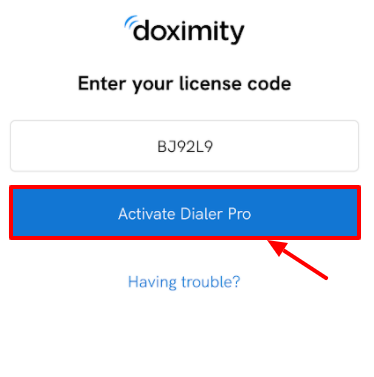This is a detailed section of a web page with a clean and minimalistic design against a white background. At the top, there are three bold blue horizontal bands, each aligned with the letter "D" in the word "Doximity," which is prominently displayed in bold black font. Below the "Doximity" heading, there is the instruction "Enter your license code" in bold black text. Directly underneath, there is a rectangular input field outlined with a thin black border containing the text "BJ92L9" in regular black characters.

Further down, there is a conspicuous dark blue rectangular button framed by a dark red border. To the right of this button, a red arrow points towards it. The center of the button features the phrase "Activate Dialer Pro" in white text. Beneath this button, there is a hyperlink with the text "Having trouble?" displayed in bold blue, indicating further assistance. The image ends abruptly without additional content, as the left, right, top, and bottom edges are cut off.